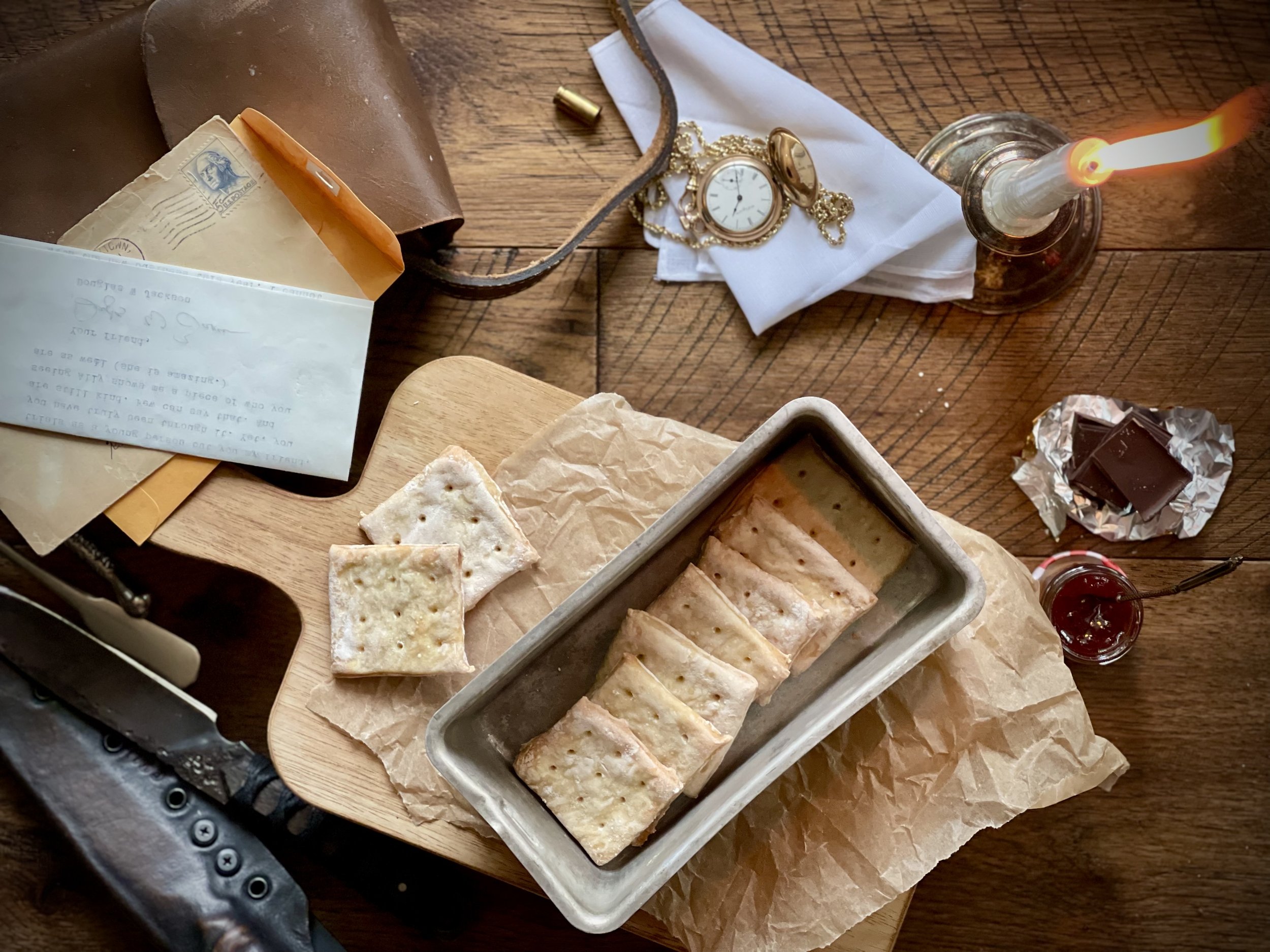The photograph captures an overhead view of a rustic brown wooden table, presenting an eclectic assortment of items. On the bottom center sits a light-colored wooden cutting board holding an oblong baking pan filled with seven golden-baked crackers, accompanied by a brown paper napkin. To the right of the cutting board, a small jar of jam rests on its lid, with pieces of chocolate wrapped in tin foil above it. The upper right corner features a brass candlestick holder with a lit white candle, casting a warm glow over the scene. At the bottom left, a sharp silver knife is sheathed beside a knife case. The upper left corner is home to a leather pouch, over which lie two envelopes, one cream-colored with a George Washington stamp, and a folded white letter. Centrally placed at the top is an antique pocket watch, adding a nostalgic touch to the setting. The table, composed of aged wooden planks, forms the backdrop, bringing a unified rustic charm to the diverse collection of items.